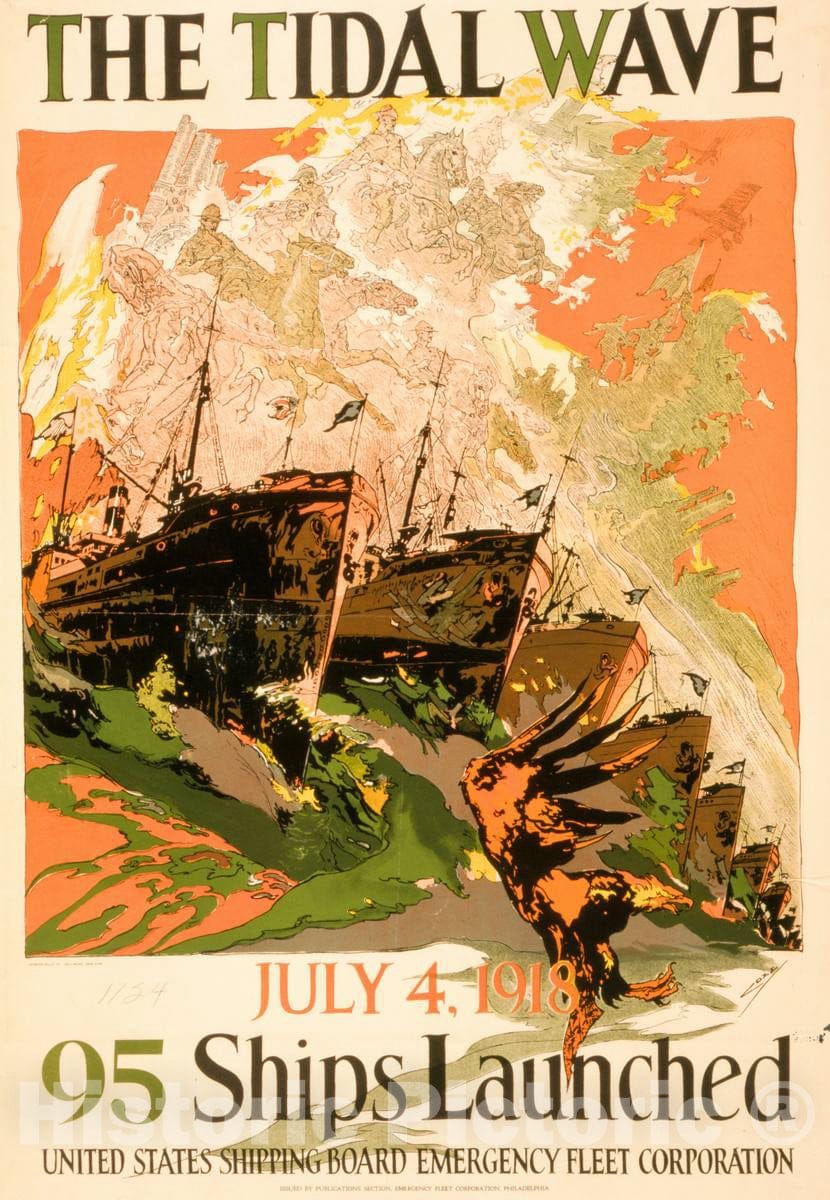This detailed and cleaned-up caption for the image is formulated as follows:

This is a detailed military poster titled "The Tidal Wave," as written in black lettering across the top border of the image. The prominent poster features a central painting of seven brown warships with masts and flags, depicted in various states of proximity from left to right, with the closest ship on the left side, and the farthest ships appearing smaller and more distant on the right, giving a sense of depth and distance. The ships are navigating through tumultuous green and beige waters, and the sky above them is colored with a vivid orange background, interspersed with smoke in hues of brown, pink, white, and yellow. The scene suggests a dramatic, almost dream-like quality as if the ships are in a troublesome battle at sea. The outer border of the poster is pink, and within it at the top, the title "The Tidal Wave" is clearly visible. The lower section of the pink border contains important historical text in orange lettering: "July 4, 1918," marking a significant date. Just below this, in bold black letters, it states "95 ships launched" and continues with a smaller inscription, "United States Shipping Board Emergency Fleet Corporation," highlighting the poster's association with a crucial wartime maritime event.